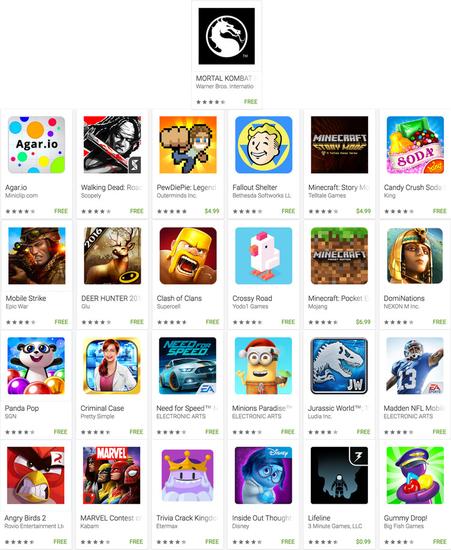This image is a screenshot of an application page displaying a variety of game apps, set against a white background. At the top of the list, you can see "Mortal Kombat." Following this are various games arranged from top to bottom: "Agar.io," "Mobile Strike," "Panda Pop," "Angry Birds Epic," "Walking Dead: Road to Survival," "Deer Hunter 2016," "Criminal Case" (featuring a woman in a lab coat), "MARVEL Contest of Champions" (showcasing Wolverine, The Flash, and Spider-Man), "PewDiePie's Tuber Simulator," "Clash of Clans," "Need for Speed," "Trivia Crack Kingdoms," "Fallout Shelter," "Crossy Road," "Minions Paradise," "Inside Out Thought Bubbles," "Minecraft: Pocket Edition," "Jurassic World," "Lifeline," "Candy Crush Soda Saga," "DomiNations," "Madden NFL Mobile," and "Gummy Drop!" (featuring a gummy bear cop holding other gummy-shaped items). This page is designed for users who have not yet installed these games or are browsing to find new gaming applications to download.